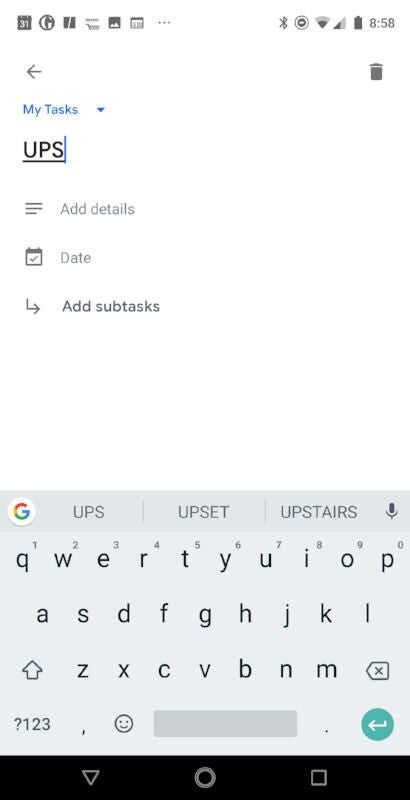This is a detailed screenshot of a Notes app or a task management application on an Android device. The top left corner features a series of gray icons, including a calendar with the date "31", a white "G" inside a gray circle, a gray box with a line through it, an indistinguishable fourth icon, a picture or gallery icon, and a clock. Additional icons include three dots indicating more options.

On the top right, there are more gray icons for Bluetooth, Wi-Fi, service strength, battery level, and the time, which reads "58". There is also a trash can icon, possibly for deleting tasks.

The main section of the screenshot is titled "My Tasks" in blue, with a downward arrow suggesting it can be expanded or collapsed. Under this, there is a task labeled "UPS" presumably entered by the user. Below the task are clickable options to "Add details, date" or "Add subtasks", allowing for further customization or expansion of the "UPS" task.